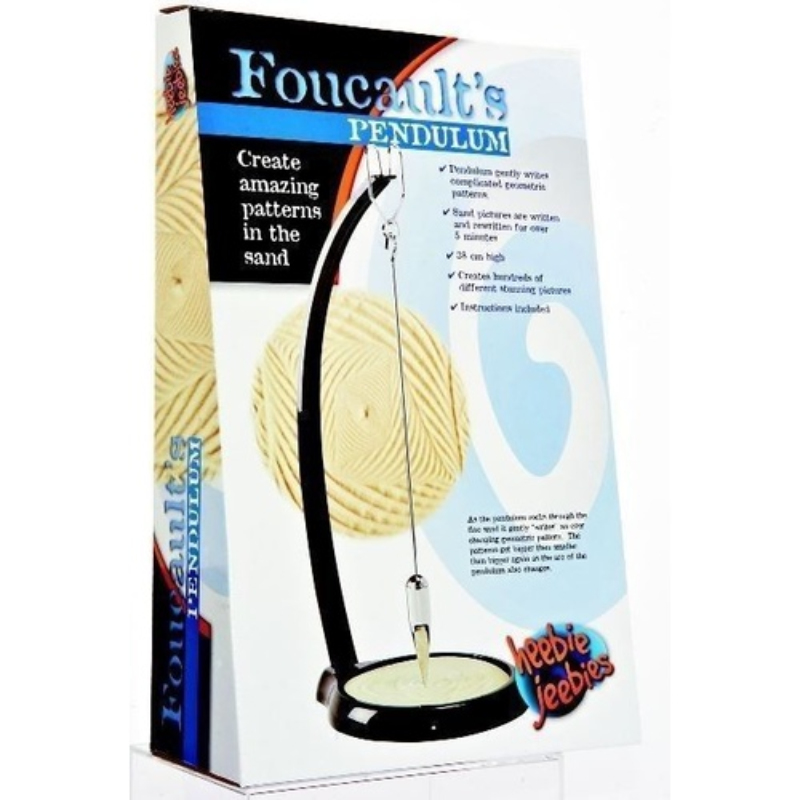This box contains a fascinating pendulum device titled "FOUCAULT'S Pendulum," prominently displayed in light blue letters, with "PENDULUM" written beneath in a blue banner. The box features an image of a pendulum suspended from a black and pale yellow base, with a crystal hanging from a metal hook, poised to create intricate sand patterns. The background is a mix of blue, white, and black colors, with a backdrop of sand that appears to be shaped by the pendulum itself. The front of the box includes the description "Create amazing patterns in the sand" and mentions that the pendulum "gently writes complicated geometric patterns" which can be "written and rewritten forever, for over five minutes." An additional note describes it as "thirty-eight centimeters high" and capable of creating "hundreds of different stunning pictures," with instructions included. Although some of the text on the right side of the box is blurry and difficult to read, the logo at the bottom right in blue and orange lettering unmistakably states "heebie jeebies," indicating the brand or maker of this intriguing tool.